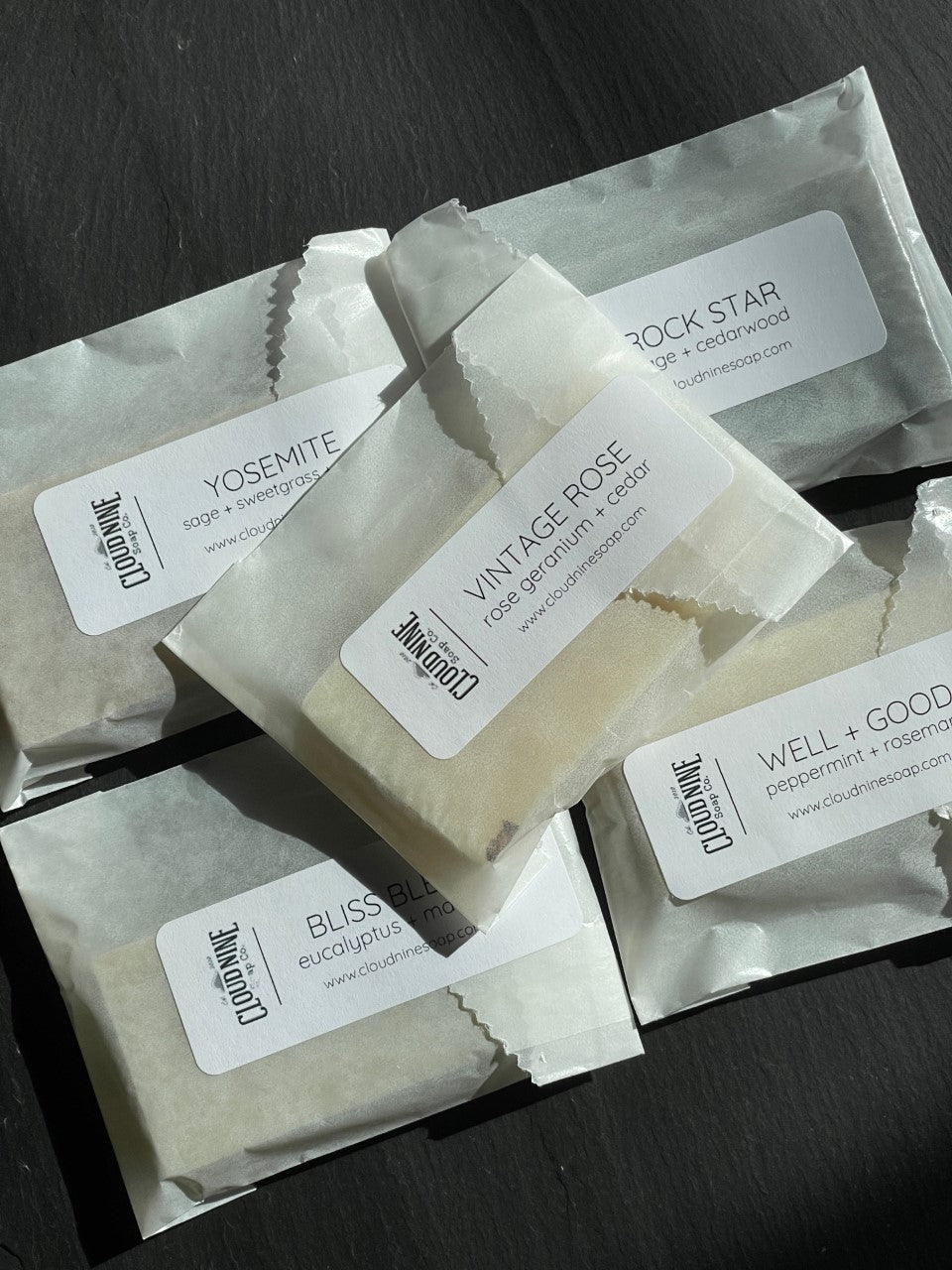In the photograph, five wax-paper-sealed bars of soap are meticulously arranged on a black wooden countertop. These soaps are presented in semi-translucent white wax bags, each featuring a prominent white sticker that secures the flap closed, ensuring the product remains enclosed. The packaging displays the brand name "Cloud 9 Soap Co.," with the web address www.cloud9soap.com visible on each label. The soaps are arranged with four at the bottom and one positioned diagonally on top. Each bag is labeled with a scent name in capital letters and details on the fragrance ingredients.

The scents are as follows:
- "Yosemite," which combines Sage and Sweetgrass, located at the bottom left.
- "Rockstar," featuring Sage and Cedarwood, placed to the bottom right.
- "Vintage Rose," blending Rose Geranium and Cedar, is the diagonally positioned top soap.
- "Bliss," showcasing Eucalyptus and an obscured secondary ingredient, found on the bottom left.
- "Well and Good," with the refreshing mix of Peppermint and Rosemary, located at the bottom right.

The arrangement and detailed labeling highlight the natural and wholesome ingredients used in these luxurious soap bars by Cloud 9 Soap Co.